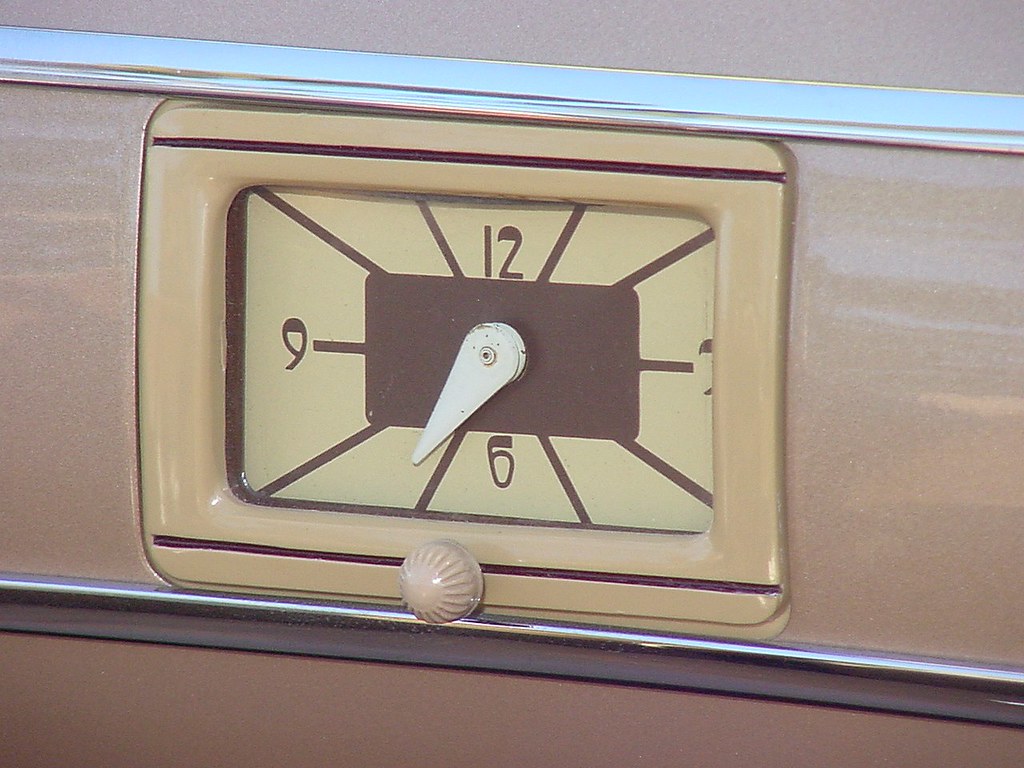This image depicts a sophisticated wristwatch with a square face. The watch face features a minimalist design, with only the 12, 3, 6, and 9 numerals displayed, leaving the other positions marked by distinct, long brownish lines. The single visible hand on the dowel is white, complementing a white button used for setting the time. The outline of the watch face is off-white, accented by a brown stripe running horizontally across the top and bottom. The band, which appears to have a glassy finish, is adorned with a turquoise blue outline on its upper side, adding a touch of elegance and modern flair to the timepiece.